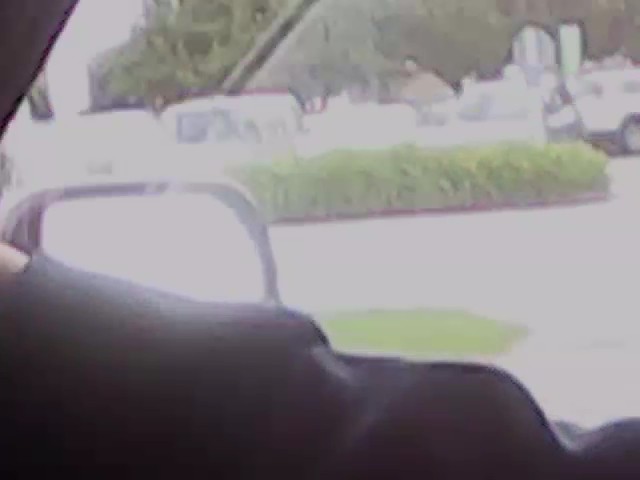This image captures a scene from the interior of a moving car, evidenced by the blurred quality of the photo. In the foreground, there's a noticeable clothed arm or leg adorned in dark fabric, hinting at the presence of a passenger. Just above this, the car's side view mirror is visible. The window beside the mirror appears to be partially open, offering a view of the outside. Through the window, a parking lot comes into sight, featuring several parked cars aligned near a row of shrubs. Beyond the parked cars, a cluster of large, green trees stands out against the background. The overall image is blurred, with colors appearing muted and less vibrant.